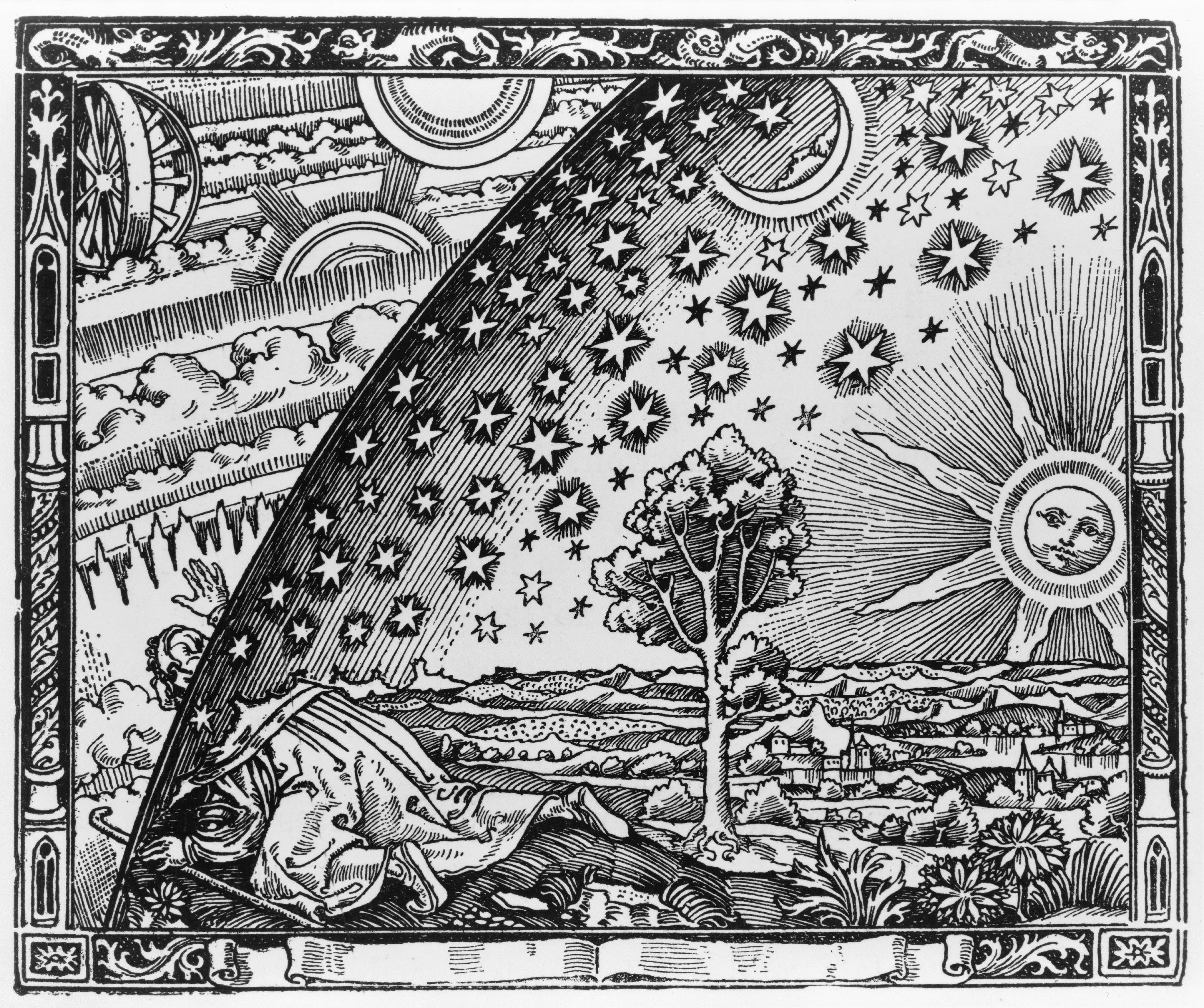This intricate and busy black-and-white illustration is bordered with elaborate scrollwork and ancient-inspired designs. The artwork features a diverse array of elements, carefully detailed to captivate the viewer. In the lower-right corner, a small piece of land is depicted, adorned with trees, flowers, and lush plants. A figure lies prone on the ground, partially obscured from view. This person is dressed in a long cloak or gown, holding a cane in their left hand, and their pointed shoes are visible. 

To the right of this figure stands a solitary tree that grabs attention amidst the lower scene. Dominating the right side of the illustration is a stunning depiction of the sun, characterized by a face with expressive eyes, a prominent nose, and a serious mouth at its center. Surrounding the sun are meticulously drawn lines and an array of stars. Additionally, a crescent moon, also with a facial expression, rests above this celestial arrangement. In the upper-left corner, the illustration is completed with the inclusion of two wagon wheels, adding an unexpected yet intriguing detail to this profoundly detailed masterpiece.